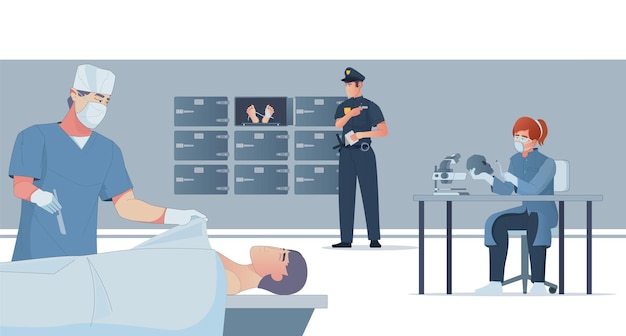The illustration depicts a detailed scene inside a morgue. At the center, a doctor dressed in scrubs and wearing a mask is holding a scalpel and appears to be performing a surgery or autopsy on a man lying on a table, his body covered with a blue sheet. To the left, a backdrop reveals a morgue wall with multiple grayish-blue compartments, one of which is open and shows the exposed feet of a body. Standing beside this morgue area is a police officer in uniform, holding a notepad and observing the scene. On the right side of the image, a woman with red hair, also in scrubs and wearing glasses, is seated at a table. She is examining a skull with intense focus, aided by a microscope-like instrument on her desk. The intricate details, from the medical instruments to the expressions on the characters' faces, convey a meticulous forensic examination in progress.